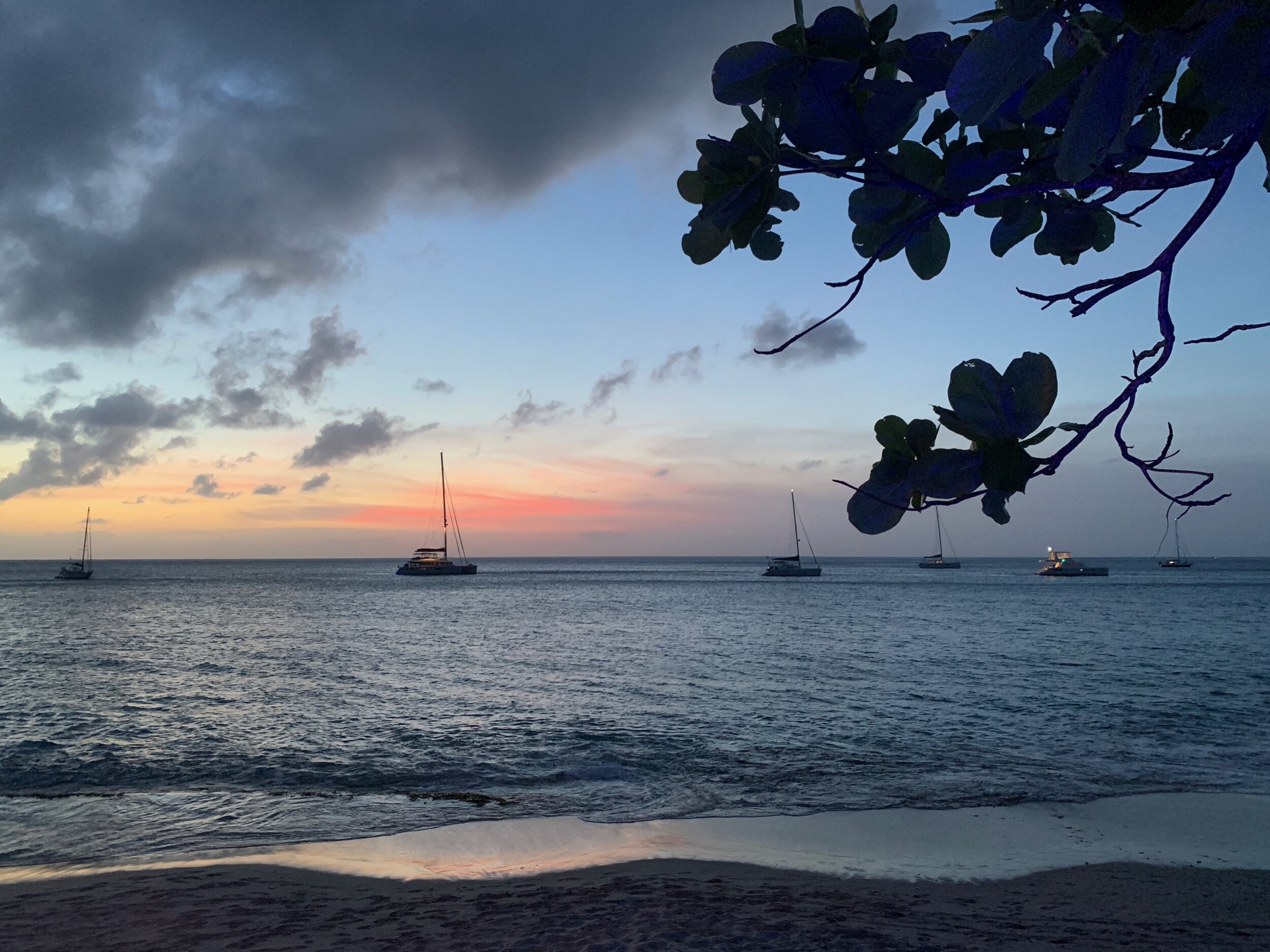A serene photograph captures six anchored sailboats near the shoreline under an ambiguous sky, likely during either sunrise or sunset. The overall coloring is muted, presenting a steel blue ocean and a gray sky, with hints of orange light peeking through the clouds closer to the horizon. Heavily gray clouds dominate the upper left corner, providing a dramatic backdrop. The calm, still water reflects the tranquil ambiance as the sailboats rest with their sails lowered, their masts highlighted against the gradient evening sky. In the upper right corner of the foreground, a silhouetted tree branch with leaves barely visible adds a natural frame to the image. The scene also includes a subtle beach with sand in the foreground, enhancing the peaceful maritime setting.